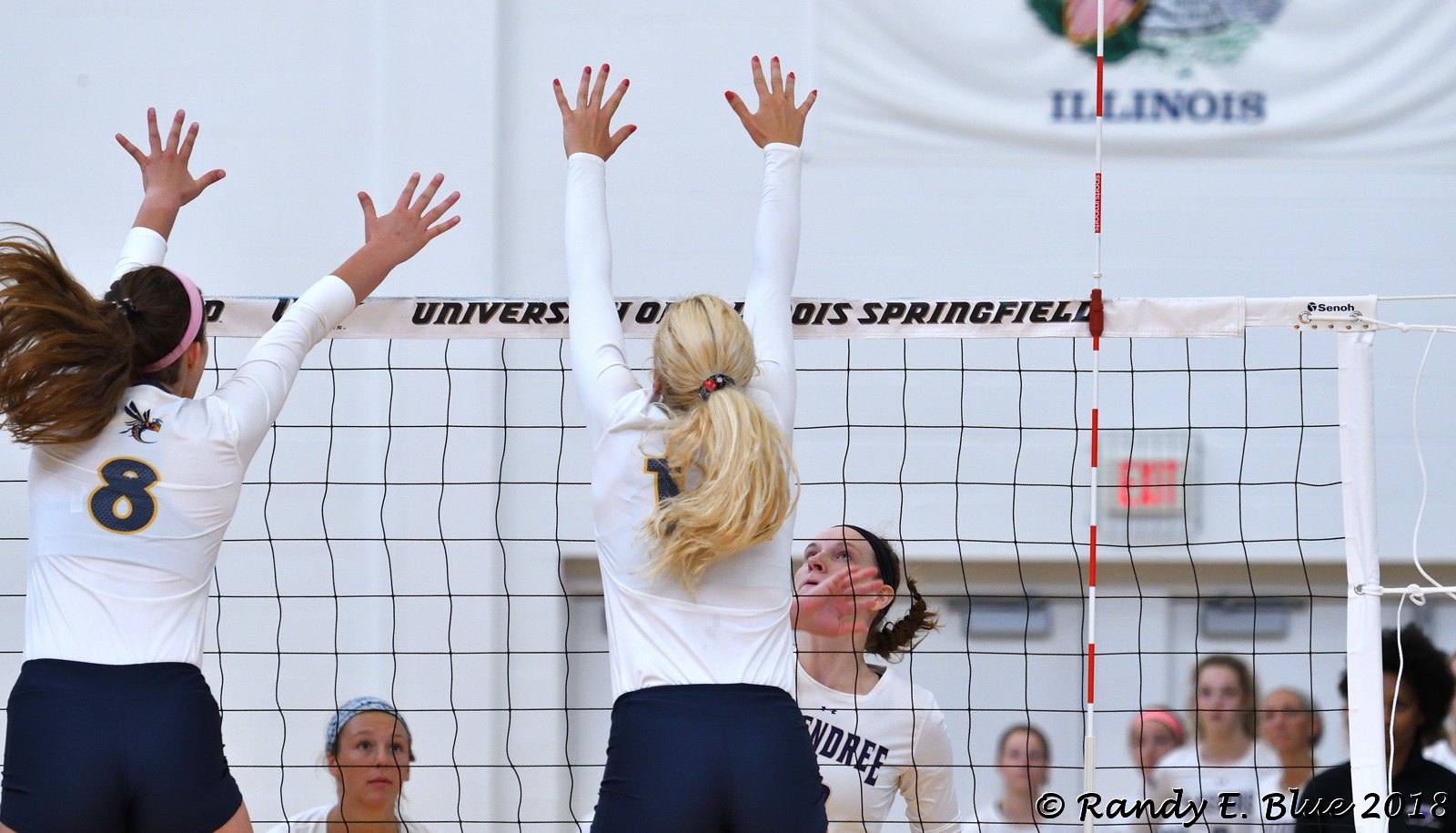This dynamic image captures an intense moment in a women's volleyball game. At the forefront, two female athletes are captured mid-jump, preparing to block a volleyball coming over the net. Both women are clad in white tops with blue shorts, their jerseys featuring blue numbers trimmed in yellow. The player on the left, sporting the number 8 and a pink headband, has dark hair, while her teammate to the right has blonde hair and can only partially reveal her number due to her hair blocking it, possibly showing a '1'. Notably, the blonde player is wearing red fingernail polish. The court is set indoors at a stadium adorned with a white banner that reads “ILEONIAS” and bearing a symbol for an exit door. The net prominently displays the University of Illinois Springfield branding. In the background, several figures, likely fans and possibly some players, are blurred, contributing to the onlookers' lively atmosphere. The photograph is dated with a small inscription at the bottom left corner reading "Randy E. Blue, 2018," adding a professional credit to the captured moment.